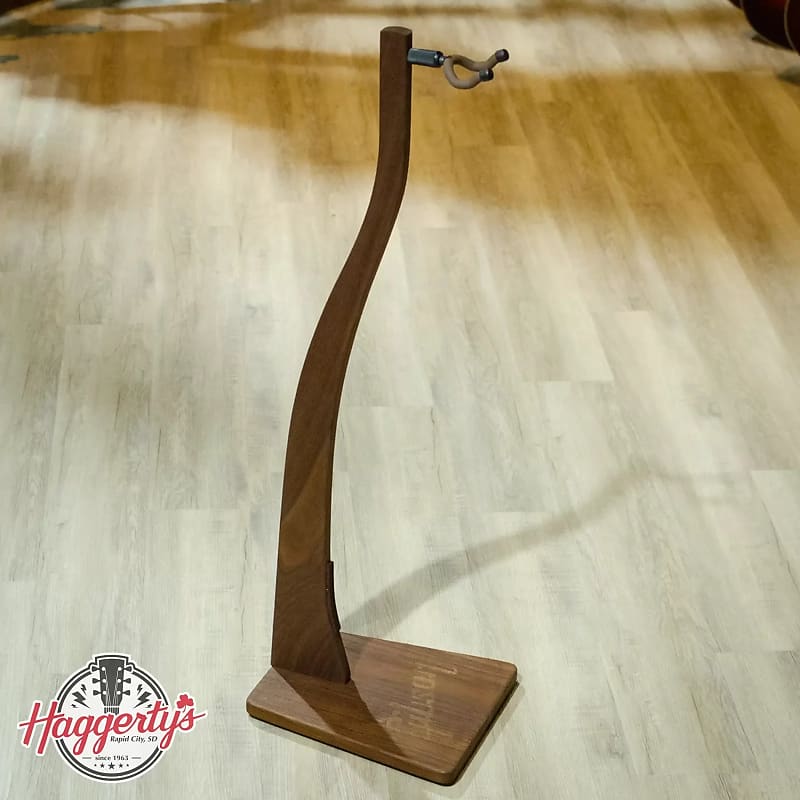The photograph features an old-fashioned wooden guitar stand positioned on a light hardwood floor. The stand comprises a flat, square wooden base marked with the word "Gibson" in gold lettering. Ascending from the base is a tapered, curved wooden support culminating in a metallic two-pronged fork designed to hold a guitar. On the bottom left corner of the image, there is a circular logo showing a guitar head with lightning bolts, adorned with red text reading "Haggerty's" and smaller black text underneath that states "Rapid City, SD" followed by "since 1963" alongside some stars. The overall scene appears meticulously arranged and possibly intended for a store display.